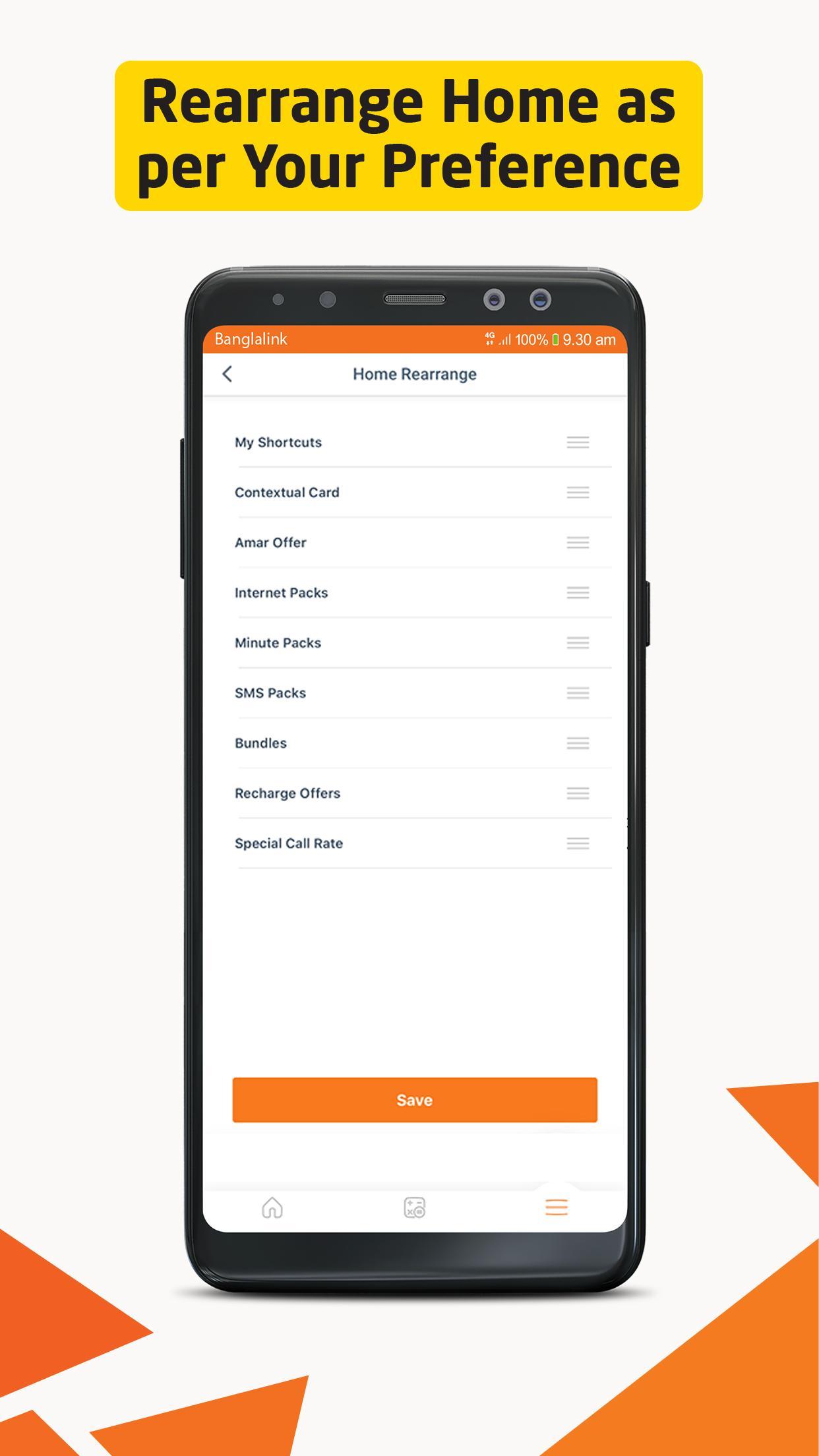The image features a predominantly white background with a yellow box at the top displaying bold, black letters that read, "Rearrange Home as per your preference." Below this box, an image of a black iPhone, approximately 6 inches in size, is depicted. The phone's screen shows a user interface with various menu elements.

At the top of the phone screen, there is an orange banner that reads "Bangalink." Beside it is the battery indicator showing 100% charge (930mAh) and a high 4G signal strength. Below this, the main section of the screen has a white background with the title "Home Rearrange" centered at the top.

The menu options are listed vertically in black text on the left side, which include:
1. My Shortcuts
2. Contextual Card
3. AIMER Offer
4. Internet Packs
5. Minute Packs
6. SMS Packs
7. Bundles
8. Recharge Offers
9. Special Call Rates

To the right of each menu option are three horizontal lines, indicating a dropdown menu for each item.

Below the menu options, there is a blank white square, which is followed by a button labeled "Save" with an orange background and white text. At the bottom of the phone screen, there are icons for the home, images, and another menu represented by three lines.

The lower portion of the image outside the phone displays an abstract background with random orange triangles set against a white backdrop, encircling the white center of the image.